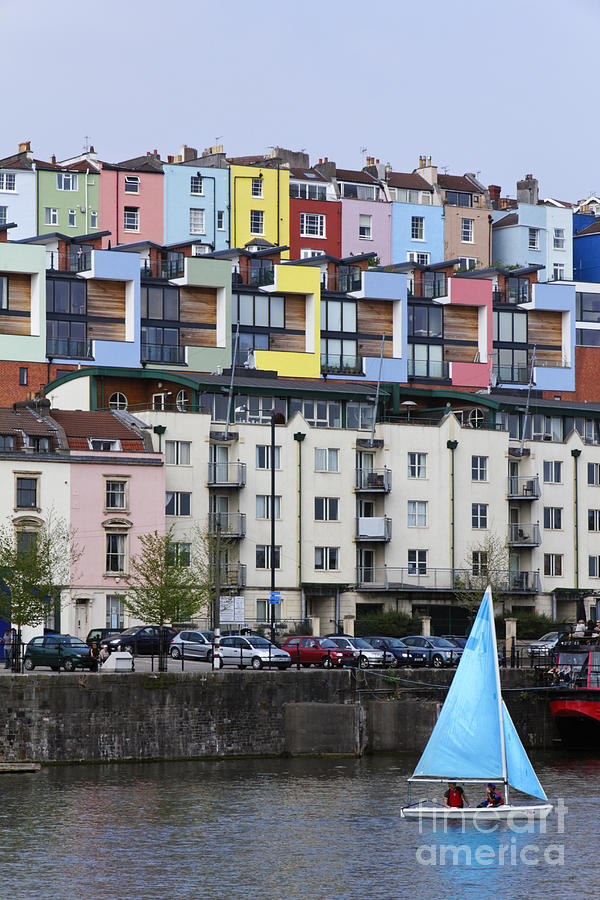The photograph captures a vibrant scene of a canal lined with a variety of colorful buildings, as seen from water level. In the foreground, a small white sailboat with a bright blue, triangular sail navigates the dark waters, reflecting the boat and surrounding structures. Two individuals aboard the boat are wearing red life jackets. The canal is separated from a parking lot by a dirty, brownish-gray brick wall. The parking lot is filled with numerous cars.

The buildings ascend in a layered architectural style, starting with a row of four-story buildings at the bottom, marked by their tan exteriors and balconies, save for one pink building. Above this layer, an eclectic mix of pastel-colored structures, sporting wood detailing and large windows, adds a splash of vibrancy. These buildings are painted in hues of green, blue, yellow, and pink. Capping the scene are even more colorful buildings, each with two large windows and painted in an array of colors including green, pink, blue, yellow, red, purple, and tan. In the bottom right corner of the image, a watermark reads "Fine Art America," adding a subtle text overlay. The overall impression is one of a lively, picturesque waterfront community with a distinct, multi-hued charm.